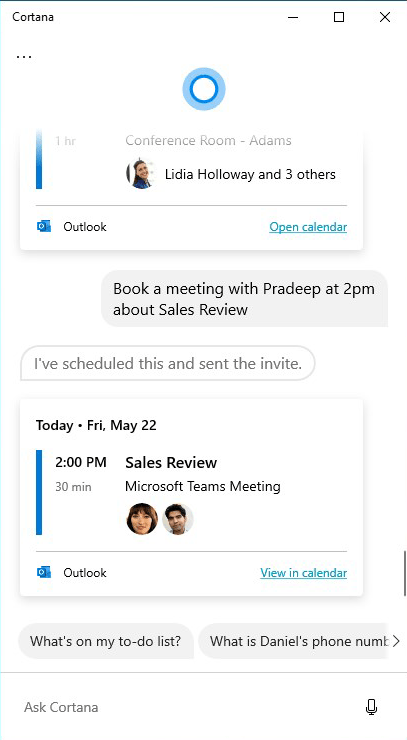This is a detailed screenshot capturing the interface of Cortana, the voice assistant integrated into Windows PCs and laptops. The interface appears as a compact dialogue box, resembling an open message window. At the top-left corner of the box, the title "Cortana" is displayed, while the top-right corner hosts the window control icons to minimize, maximize, and close the window.

Directly below these controls, a small, glowing blue circle indicates active communication with Cortana. The main visible message appears to be a reminder from Cortana, stating: "Conference room: Adams, Lydia, Holloway, and three others." An Outlook icon is situated to the left of this reminder, and an "Open calendar" option is on the right.

Beneath the reminder, user interaction is shown. The user has instructed Cortana to "book a meeting with Pradeep at 2 p.m. about sales review," to which Cortana responds, "I've scheduled this and sent the invite." Following this exchange, a confirmation details the meeting: "Today, Friday, May 22, 2 p.m., a 30-minute meeting, Sales review, Microsoft Teams meeting." An icon of two people, likely representing the user and Pradeep, is displayed beside this confirmation.

Following this are two options for the user to continue the conversation: "What's on my to-do list?" and "What is Daniel's phone number?" Finally, at the bottom of the screen is the message box for typing responses to Cortana. To the right of this box, there's a small microphone icon for recording voice messages.